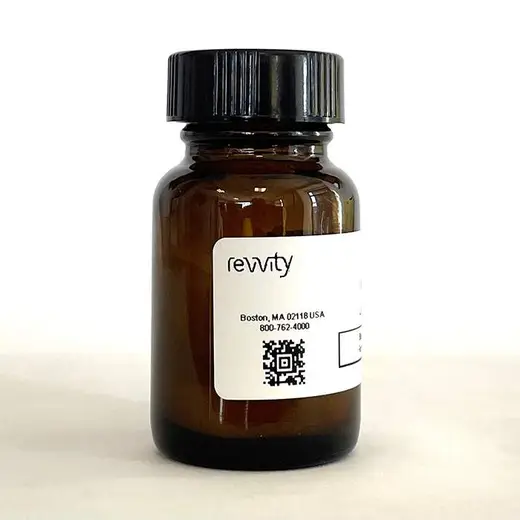This photograph features a squatty, dark brown glass bottle with a black, child-safe cap that has vertical ridges. The bottle is sitting on a cream-colored table or countertop against a white wall, creating a very simple and clean aesthetic. The bottle has a white label on its front, which prominently displays the word "Revity" at the top, spelled as R-E-V-I-T-Y. Below this, the label reads "Boston, MA 02118 USA," followed by a phone number, "800-762-4000." Further down, there's a QR code for additional information. The label wraps around the bottle slightly, revealing an unreadable square on the right side. The general consensus is that the bottle appears to contain medication or a high-end cream.